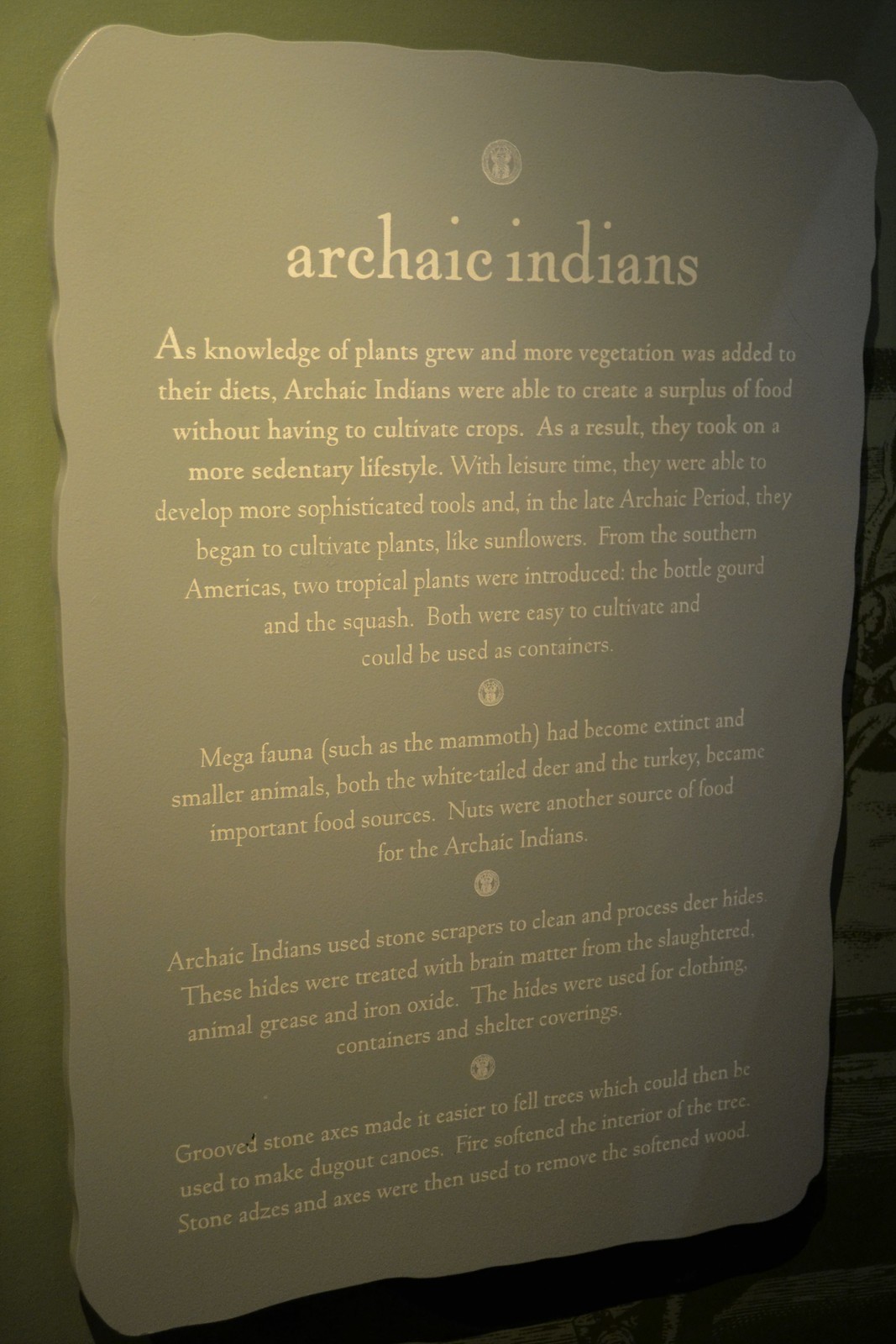The image depicts a museum plaque styled to resemble an ancient stone tablet, evoking the imagery of Moses' Ten Commandments with its roughly hewn and weathered edges. Hanging against a dark green or stone-brown background, the plaque is inscribed with yellow text. At the top center, it reads "Archaic Indians." Below this heading, the text describes the lifestyle and innovations of the Archaic Indians. 

As their knowledge of plants expanded, the Archaic Indians incorporated more vegetation into their diet, allowing them to create food surpluses without the need for crop cultivation. This led to a more sedentary lifestyle, where they had the leisure time to develop sophisticated tools. In the later Archaic period, they began cultivating plants like sunflowers from Southern America and introduced two tropical plants—the bottle gourd and the squash—both of which were easy to cultivate and used as containers.

With the extinction of megafauna such as the mammoth, the white-tailed deer and the turkey became vital food sources. Nuts also played a significant role in their diet. The Archaic Indians utilized stone scrapers to clean and process deer hides, which were then treated with brain matter, animal grease, and iron oxide. These treated hides were used for clothing, containers, and shelter coverings. Grooved stone axes facilitated tree felling, allowing the creation of dugout canoes. The process involved softening the tree's interior with fire, then using stone adzes and axes to remove the softened wood.